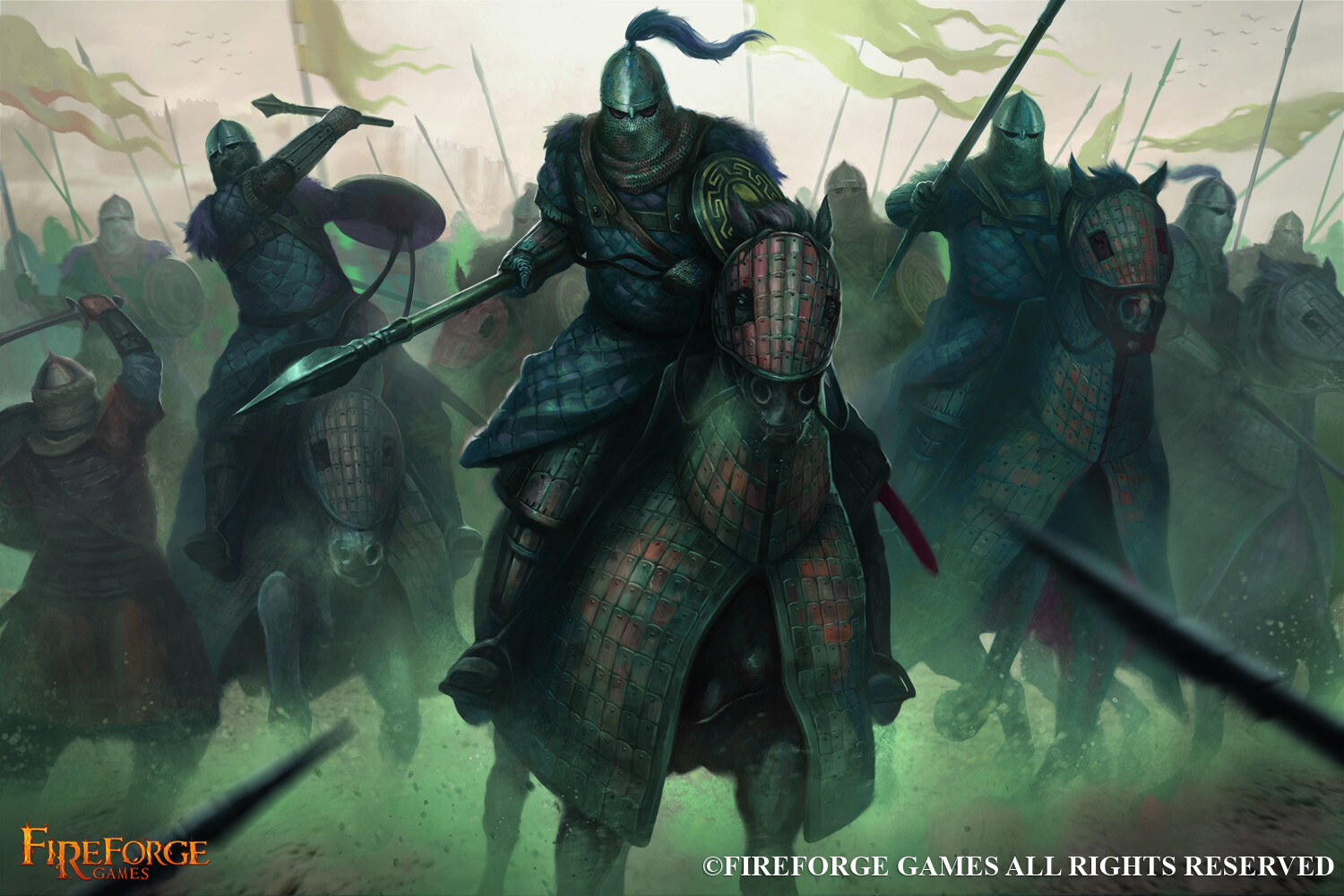This is a highly detailed image, most likely an advertisement or screenshot for a video game called "Fire Forge." The logo "Fire Forge Games" is prominently displayed in the bottom left corner in orange, while the bottom right corner features a copyright notice: "Fire Forge Games All Rights Reserved." The scene portrays a medieval battle with a formidable group of knights charging forward on horses. The central figure is a knight dressed in a blue plaid tunic, wearing a silver helmet adorned with a purple plume. He grasps a spear in his right hand and a shield in his left, charging into battle against two spears coming from the left and right sides of the picture.

The knight's helmet leaves only his eyes visible, emphasizing the intensity of the battle. His horse and shields have a greenish tint with hints of bronze and rusty brown armor. To his right, another knight rears back, ready to strike down an opponent on the ground, while to his left, a similarly armed knight also charges on horseback.

In the background, a multitude of other knights, all armored with helmets and wielding spears, prepare to charge. Above them flutter numerous flags with green streamers against a pale pink sky, suggesting unity and an organized army. Additionally, birds can be seen flying in the top right corner, contributing to the dynamic and intense atmosphere. The scene is predominantly green with occasional bronze highlights, creating a vivid and intimidating portrayal of a medieval battlefield.